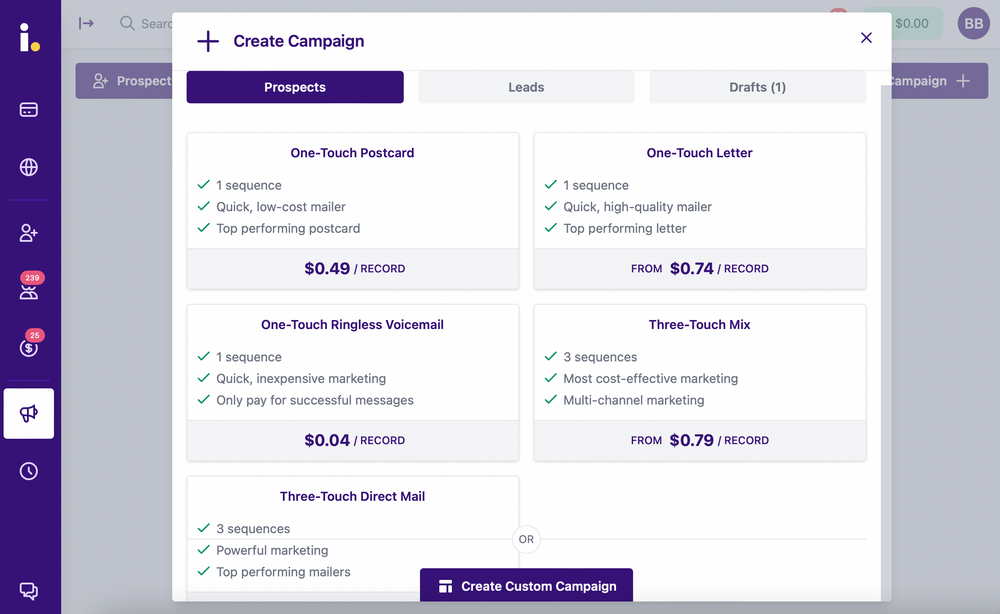The image is a screenshot of a webpage with a subdued, dark gray background. Dominating the center of the screen is a noticeable white dialog box with a header reading "Create Campaign," accompanied by a plus sign. The top of the dialog box features three clickable tabs: "Prospects" on the left, "Leads" in the center, and "Drafts" on the right, the latter of which indicates one item with a small numeral "1." 

The selected "Prospects" tab is highlighted in navy blue with white text. Below the header, there are four clearly visible boxes, arranged into two rows of two, detailing various campaign options and their associated costs. The first box reads "One-Touch Postcard," priced at 49 cents per record. The second box, titled "One-Touch Letter," is priced at 74 cents per record. The third option, "One-Touch Ringless Voicemail," costs 4 cents per record. The fourth box offers a "Three-Touch Mix," priced at 79 cents per record. 

A fifth option, labeled "Three-Touch Direct Mail," is partially cut off at the bottom of the screen, suggesting that additional information or options might be available but are not fully displayed in this screenshot.